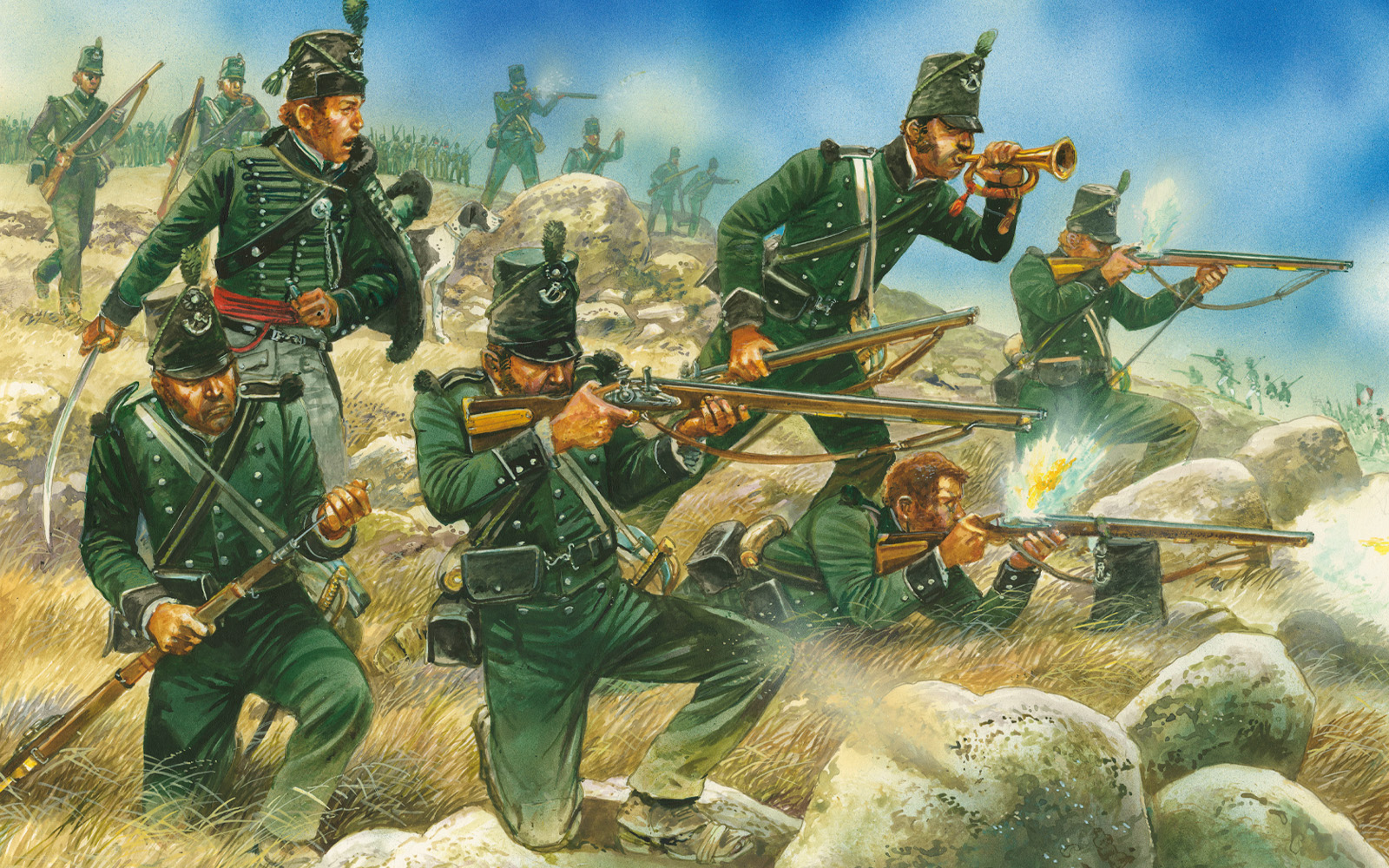The image, resembling a digital painting, depicts an intense outdoor battle scene under a blue sky with hazy clouds. In the foreground, there are six soldiers clad in dark green military uniforms with tall green hats featuring slim visors. These men are positioned amidst long brown grass and large, scattered boulders on a hillside. From left to right, the scene details:

- A soldier standing with a knife at his side, shocked expression on his face.
- Beside him, a man kneels while loading his gun.
- In the middle, a soldier is positioned aiming his rifle, flanked by another laying on the ground, his gun propped up, ready to shoot.
- Further right, another kneeling man also prepares to fire.

Dominating the center, a soldier holds a rifle in one hand and blows a bugle with the other, adding a dynamic touch to the scene. In the background, more soldiers stand in formation, though they are slightly blurred, emphasizing their distance. Among them hides a pointer dog, contributing to the realism of the battlefield setting. Together, these elements create a vivid tableau of wartime urgency and preparation.